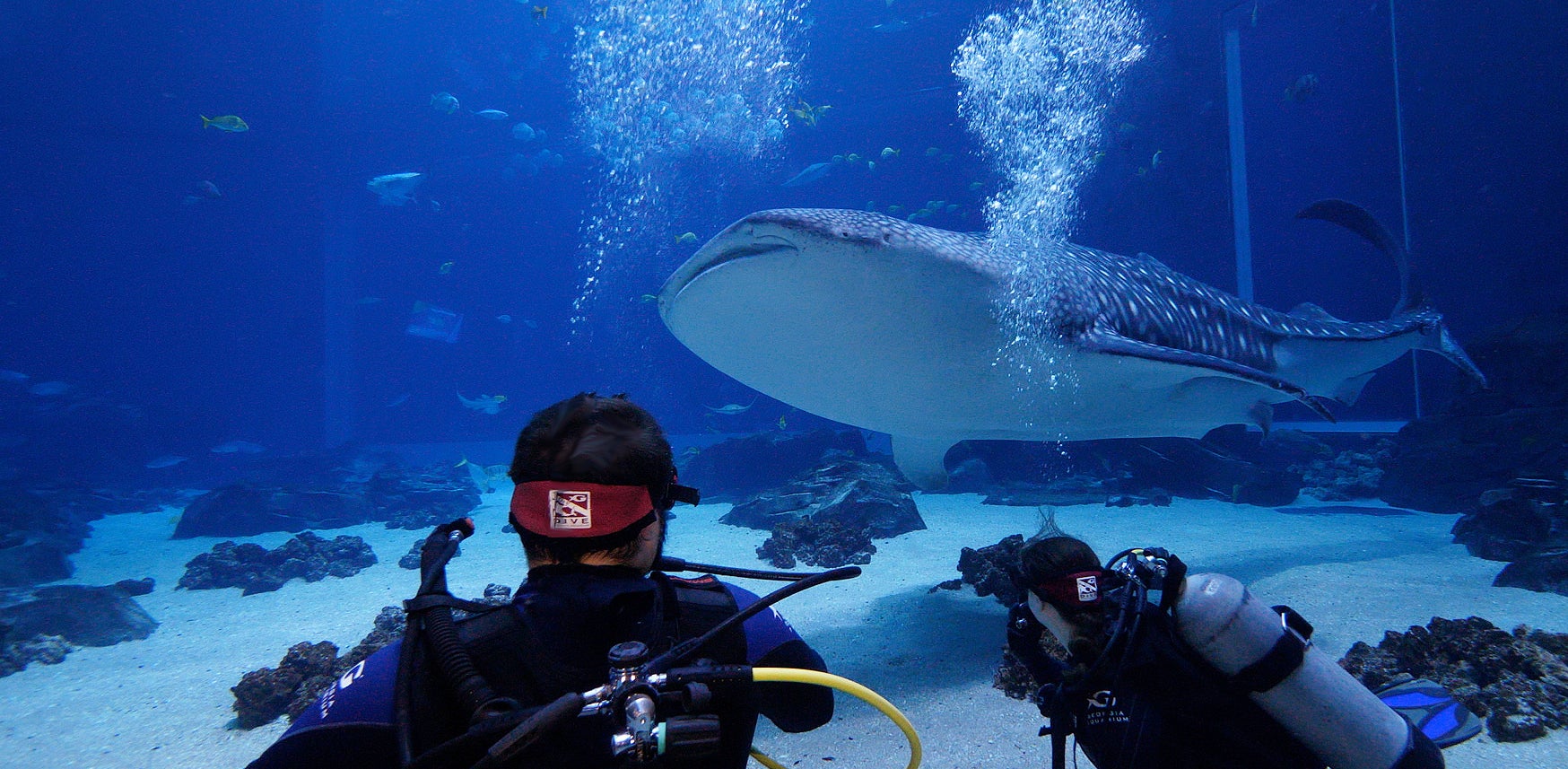In this detailed full-color underwater photograph, a pair of scuba divers are seen observing a large shark with a distinctive flat snout, commonly known to be harmless to humans. The image is horizontally rectangular with reasonably clear blue water. The bottom of the photograph features a sandy floor interspersed with black rocks and a scattering of small fish swimming around. Notably, there is an artificial, possibly plastic, rectangular structure visible in the upper right corner, suggesting that this scene might be within a controlled environment, such as a holding tank or large aquarium.

The divers are positioned with their backs to the camera. One diver, identifiable by short brown hair, is wearing a black vest adorned with various hoses and tubes linked to the gray oxygen tank he carries. Another diver appears to have a red item, possibly a hat, on their head. Sunlight penetrates from above, illuminating the scene more brightly in the center where the shark and the divers are, creating a stark contrast with the darker waters to the far right and left of the image. This interplay of light highlights the unique pattern on the shark, which has a gray body with light gray dots and a white underside.